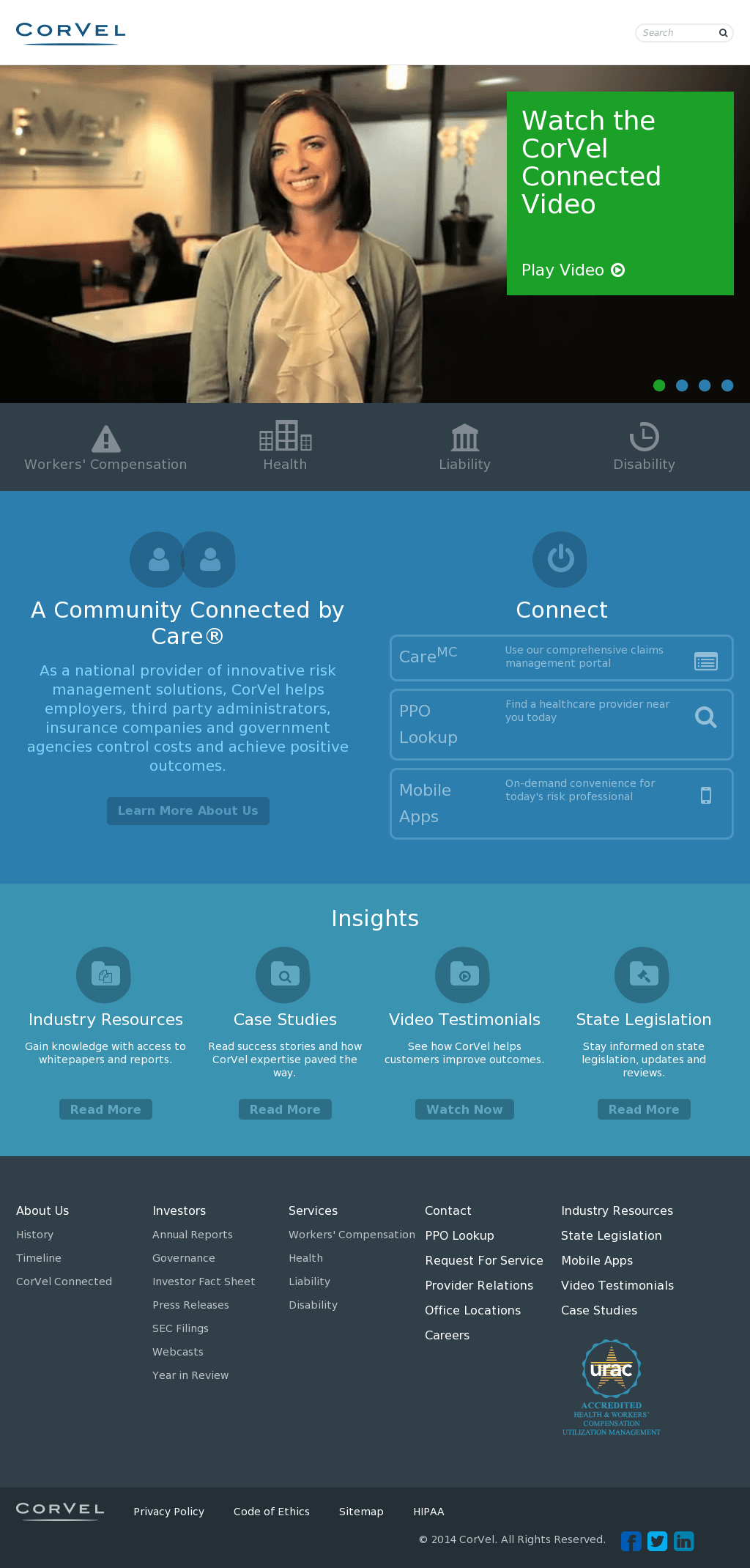In the upper left corner, the word "Corvel" is prominently displayed in blue text and underlined: "C-O-R-V-E-L". Below this, there is an image of a woman with short, dark hair, looking off into the distance and smiling. She is dressed in a white shirt coupled with a blue sweater. Behind her, a table is visible, suggesting she is in an office or business environment.

To the right of this image, inside a green square, the text reads, "Watch the Corvel Connected video," followed by "Play video" beneath it.

Below the woman’s image is a long, dark blue rectangle, followed by a standard blue square. The blue square contains the phrase, "A community connected by care," with the word "Connect" appearing to the right in white text. Below "Connect," in turquoise text, is the word "Insights," with four subcategories listed underneath in very small white text.

Towards the bottom of the layout, there is a dark blue box with five categories in very small white text. In the bottom right corner, there are three evenly spaced blue squares.